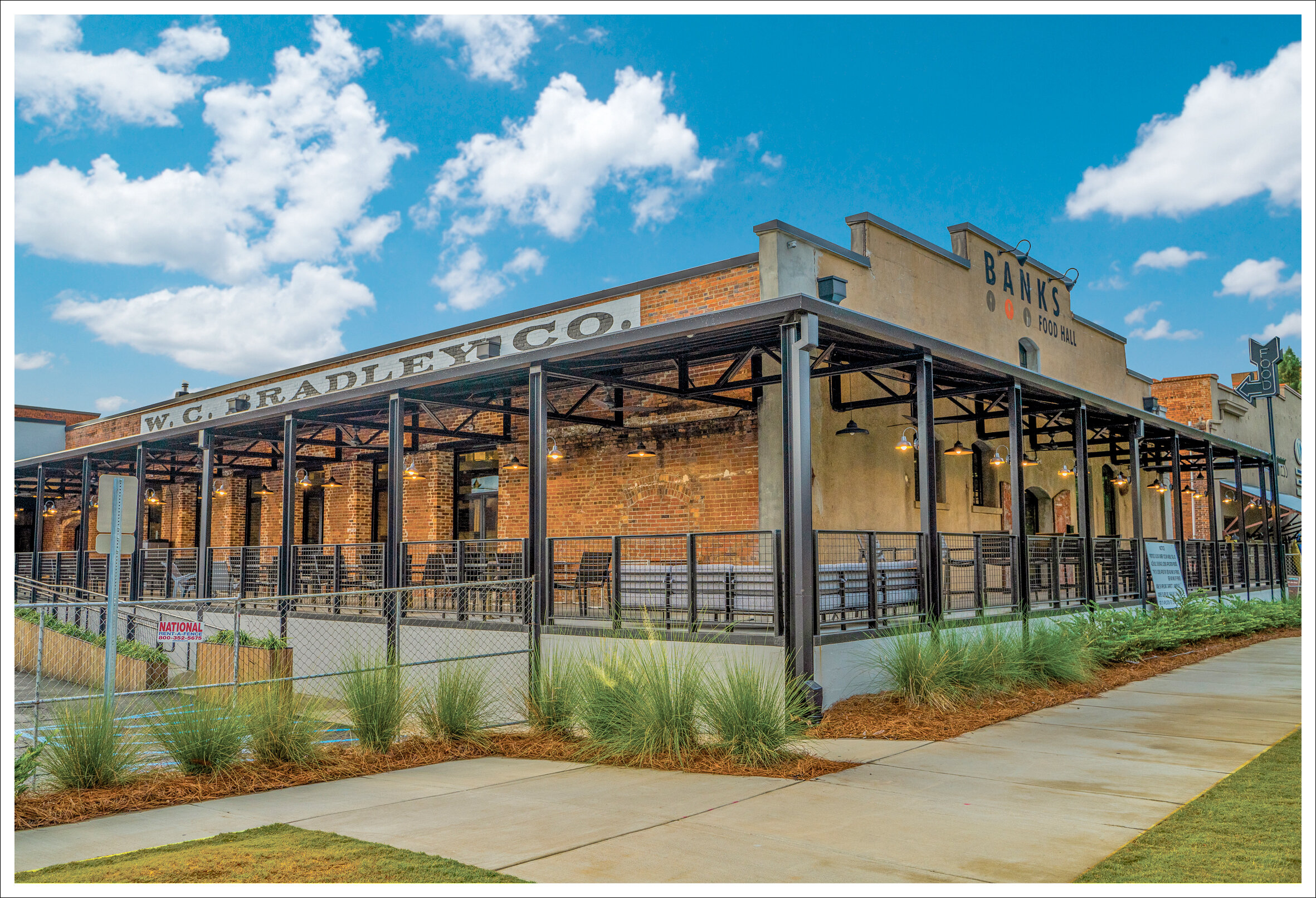The image depicts a digitally generated or three-dimensional illustration of an orange brick building characterized by its architectural style. Prominently featured is a large, horizontally oriented sign on the top of the building that reads "W.C. Radley Co." To the right, on a brown façade, the word "Banks" appears in large letters, positioned high up. Beneath "Banks," there is additional text reading "Food Hall." Vertical columns and beams frame the front and right sides of the building, and the patio is furnished. The sidewalk in front is paved and bordered by neatly planted green grass, complemented by tall grasses such as pampas grass. Overhead, a clear blue sky with white clouds completes the picturesque scene.